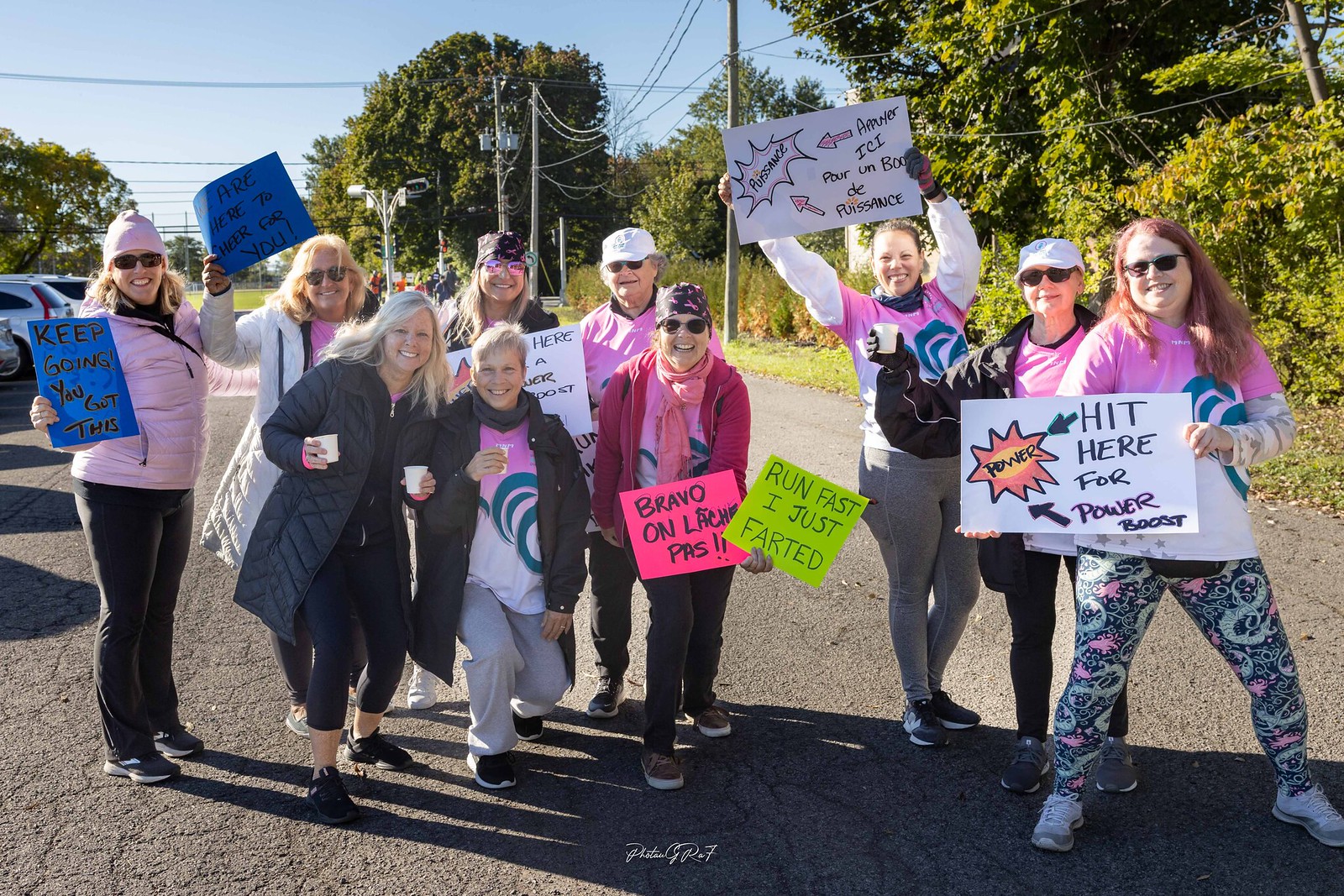In this vibrant and cheerful outdoor scene, a group of eight to ten middle-aged women, predominantly white and many wearing glasses, are standing in the middle of a cracked asphalt roadway under a bright, sunny sky. The day appears chilly, with several women donning heavy winter coats, hoodies, and hats. They all smile warmly at the camera, exuding a sense of camaraderie and enthusiasm. Each woman holds a colorful, hand-drawn poster with motivational messages, such as "Hit Here for Power Boost," "Run Fast, I Just Farted," and "Keep Going, You Got This," hinting at a fun run or a similar outdoor event. Some are also holding plastic cups, possibly containing warm beverages. The background features tall bushes and trees along the right side of the road, a line of electrical poles, and the distant outline of cars with only their rears visible. The blue sky and overall setting suggest a sense of openness and community spirit.